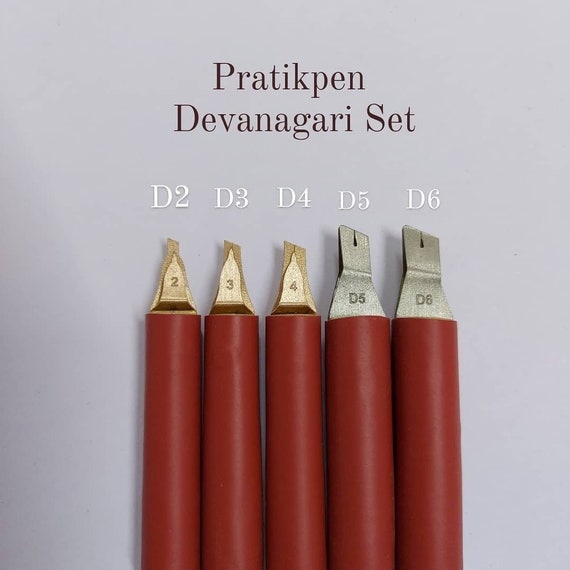This photograph showcases a Pratikpen Devanagari Set, clearly labeled at the top center in black text. The background is a subdued gray. Below the title, five meticulously arranged cylindrical tools are displayed vertically from left to right. Each tool is distinguished by both engraved numbers on their metallic tips and matching white labels overhead reading D2, D3, D4, D5, and D6.

Starting from the left, the first tool, labeled D2, features a bronze triangular tip with the number 2 embedded on it, and a maroon-colored cylindrical handle. To its right, the D3 tool has a slightly narrower bronze triangular tip with the number 3 engraved, also accompanied by a maroon cylindrical handle. The third tool, marked D4, sports a wider bronze triangular tip with a 4 etched on it and the same maroon handle.

Progressing further, the D5 tool shifts to a gray pyramid-like tip with the number D5 engraved, diverging from the previous bronze coloring. Its handle remains consistently cylindrical. The final tool, labeled D6, mirrors the style of the D5 with a gray pyramid-like tip and the number D6 etched on it, completing the set. The meticulous gradation in the size and tip shapes of each tool demonstrates an emphasis on precision and variety within the set.